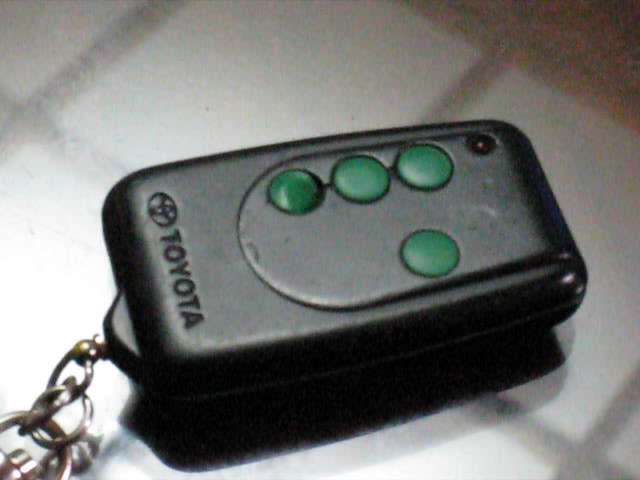This is a detailed color photograph of a Toyota car key fob taken in a close-up shot. The key fob is black and rectangular with rounded corners. Prominently displayed on the remote is the Toyota logo and the word "Toyota" in black letters, located at the bottom. There are four green buttons on the key fob: three aligned next to each other on the left, and a single button on the right. Above the three aligned green buttons is a red bubble indicator light that illuminates when any of the green buttons are pressed. The key fob is lying on a white surface with gray lines, likely a tiled floor or table, creating a pattern of white boxes. Attached to the bottom of the key fob is a keychain with silver rings, though this part is partially cropped out of the image. Additionally, the setup is such that light filters through, casting a shadow of the key fob towards the bottom right-hand side.